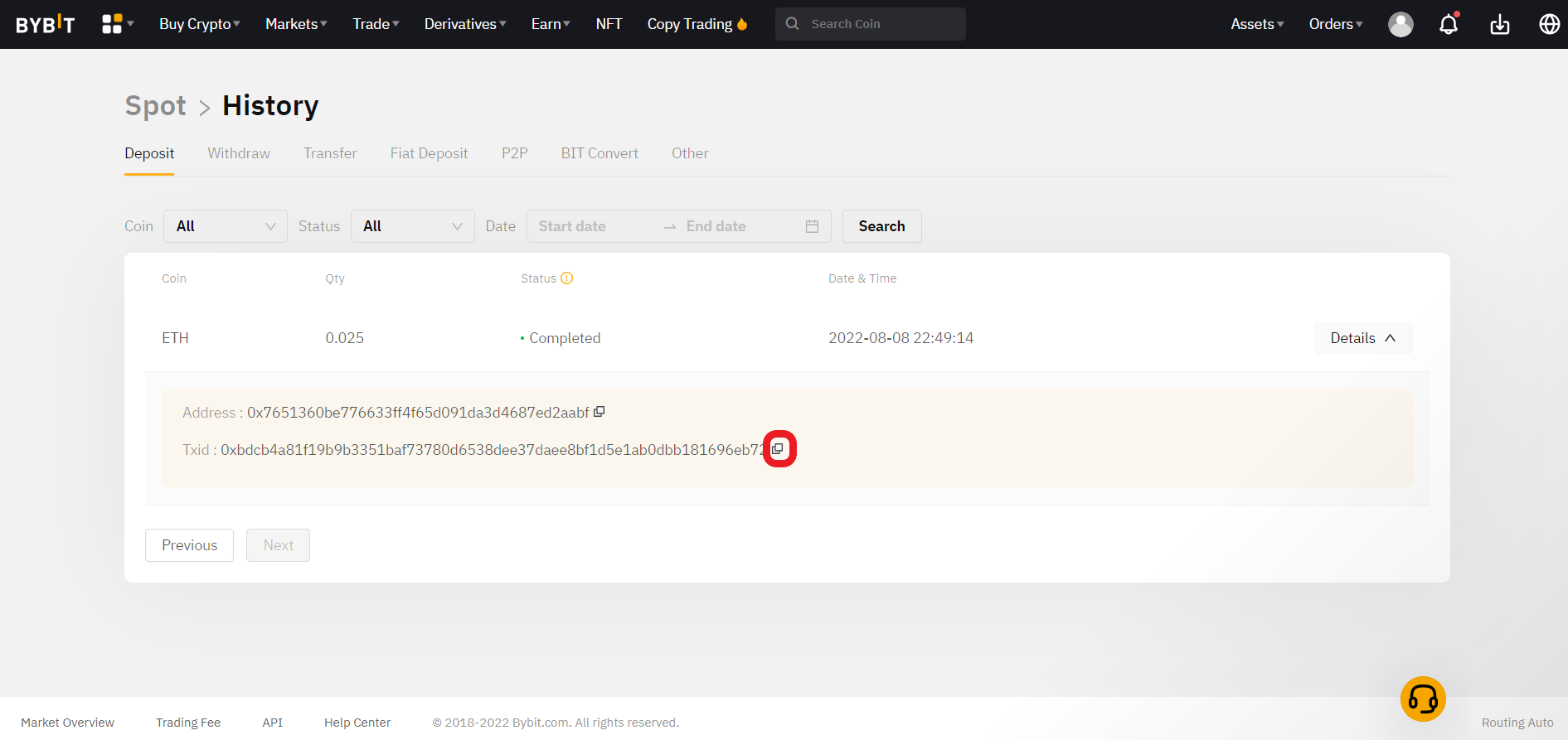**Detailed Caption:**

The image showcases a computer screen of an individual navigating the Bybit (BYBIT) website, presumably to purchase cryptocurrency. The website's brand name, "BYBIT", is prominently displayed in all caps with a distinct design feature where the letter "I" is colored in a vibrant orangey-yellow and positioned slightly above the other letters. This branding is situated on a black bar at the top of the interface.

To the right of the Bybit logo, the navigation bar includes several dropdown menus. Starting from the left, we see "Buy Crypto" in white text on the black background. Following this, there are additional dropdown menus labeled "Markets," "Trade," "Derivatives," "Earn," and links for "NFT" and "Copy Trading," the latter accompanied by a flame icon indicating its popularity or importance. Next, there's a search bar with the placeholder text "Search coin" next to a magnifying glass icon. Further to the right, the bar includes dropdown menus labeled "Assets" and "Orders," followed by an icon with the silhouette of a person representing the user profile. Additionally, there is a notifications bell with a red dot, signifying unread notifications, a download icon depicted as a box with an arrow, and a globe icon hinting at language or regional settings.

Below this top navigation bar, the main screen is visible, indicating that the user is on the 'History' page, with the word "Spot" in gray letters next to an arrow pointing towards "History." Highlighted in charcoal gray text is the option "Deposit," which is currently selected and highlighted in yellow at the bottom. Other clickable options, including "Withdraw," "Transfer," "Fiat Deposit," "P2P," "Bit Convert," and "Other," remain unselected.

Further down, there are several dropdown menus with labels like "Coin," "Status," and "Date," each offering filtering options for the displayed data. Below these filters, specific transaction details are shown: Coin is "ETH," Quantity is "0.025," Status is "Completed," Date and Time is "2022-08-08 22:49:14," with associated information about the address and TXID. Navigation buttons for "Previous" and "Next" allow users to browse through other transactions. The detailed yet streamlined layout of the screen suggests a user-friendly approach to managing cryptocurrency transactions on Bybit.